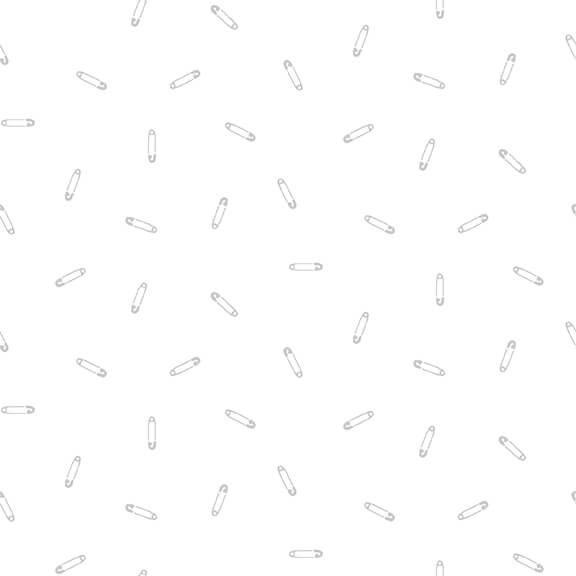The image depicts a simple yet striking pattern of small, stylized safety pins scattered across a solid white background. The safety pins, rendered in a silverish gray hue, are arranged in a repetitive triangular pattern that gives the composition a sense of organized repetition. With an estimated 40 to 70 safety pins visible, they appear to cover the entire image, though some are partially cut off by the edges of the frame. From a distance, the organized placement of these pins almost resembles sprinkles scattered over the white canvas. The clean, minimalist design makes the image suitable as a wallpaper, whether for a phone, computer, or even a decorative context.